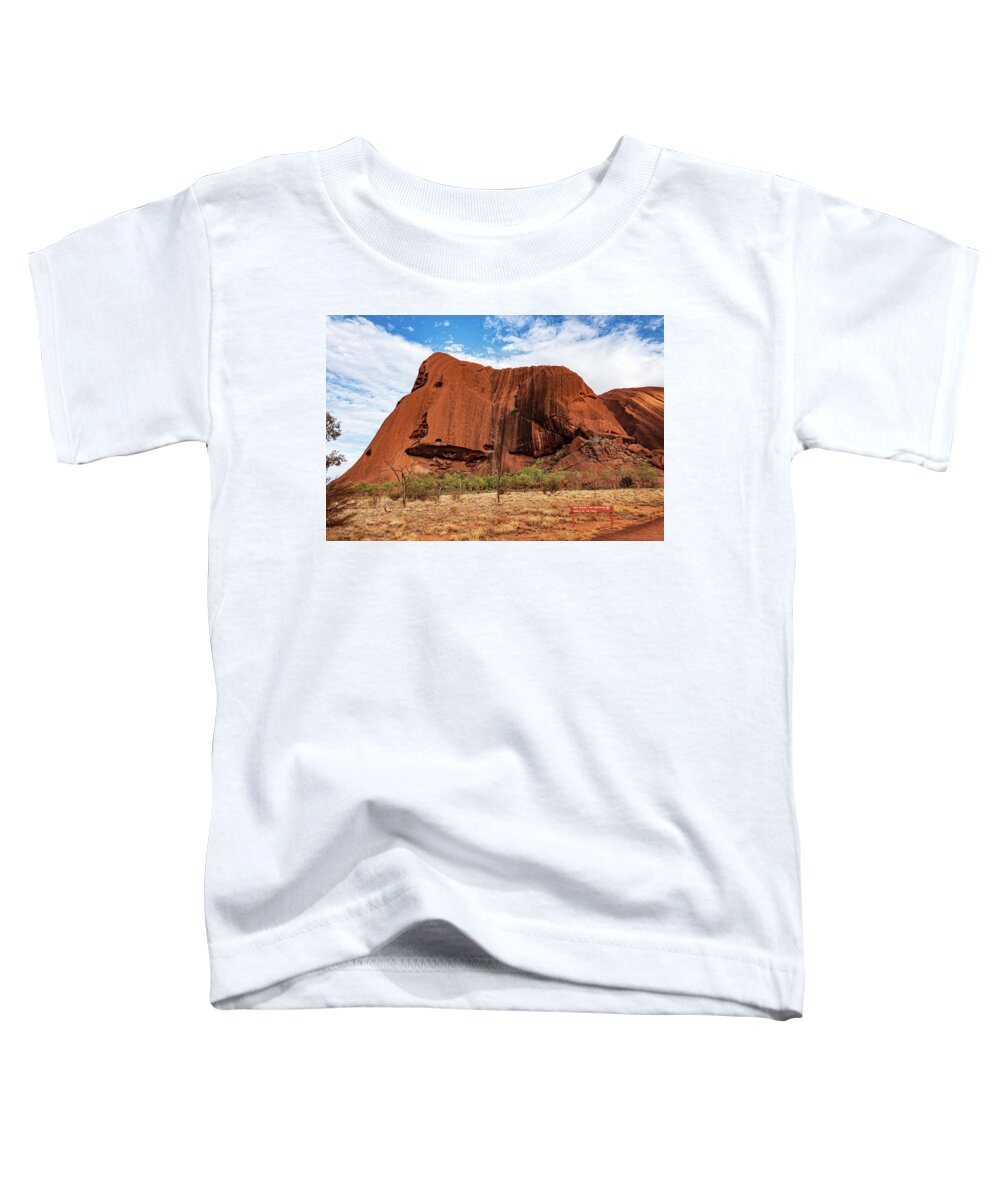The image features a white short-sleeve t-shirt with a scoop neck, laid flat against a white background. The t-shirt is slightly lifted and shows minor folds and wrinkles at the bottom. Centered on the t-shirt is a square-shaped, realistic print of a desert canyon scene. The canyon, depicted in rust and light brown hues, towers high, resembling a cliff or rock formation. In front of the canyon, the ground appears barren and a few small desert plants, including green grasses and a solitary tree on the left, are visible. The sky above the canyon is a vivid blue, adorned with numerous white clouds, indicating a daytime setting. Small details like stakes protruding from the ground enhance the realism of the landscape.